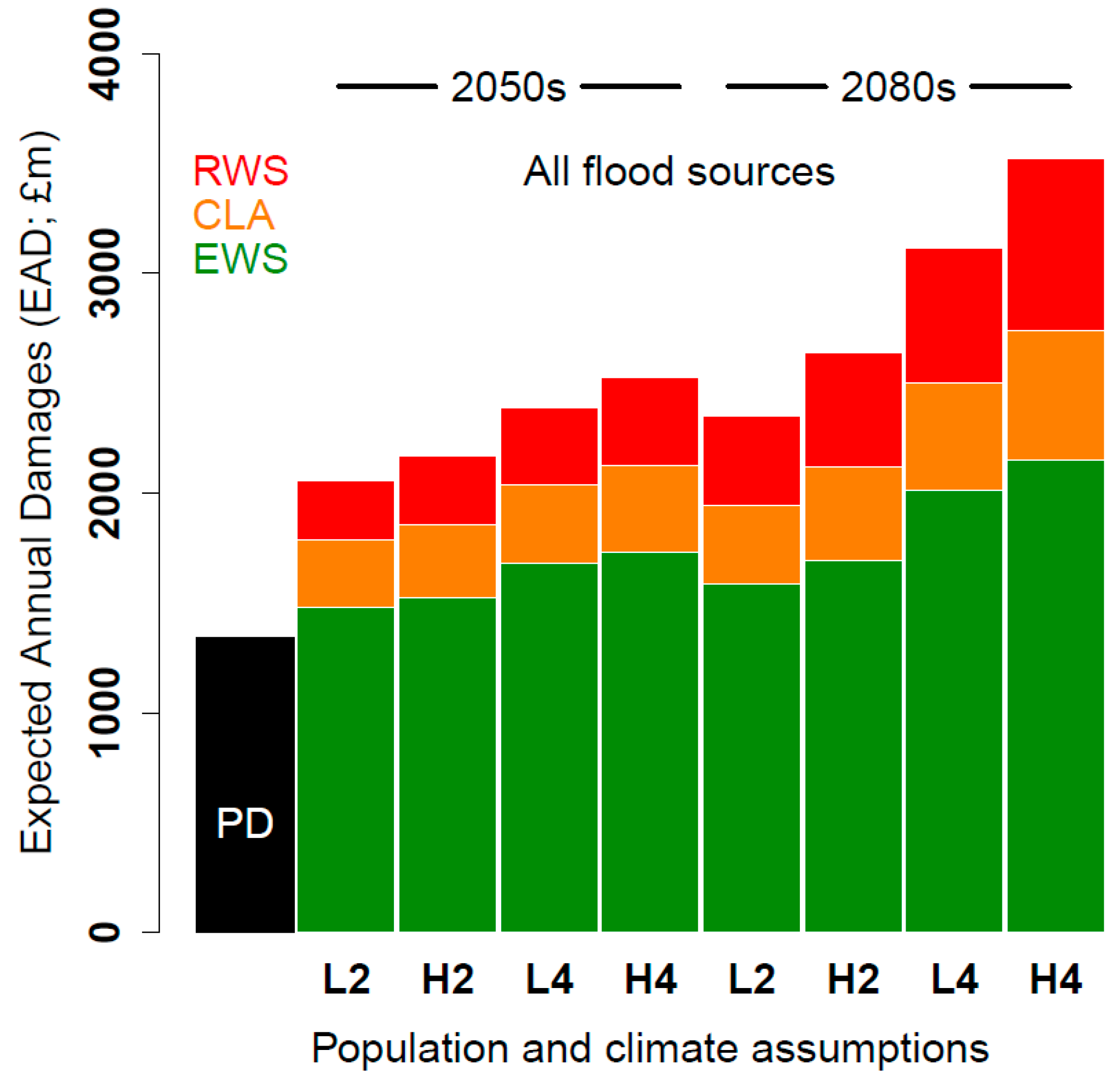The image displays a detailed bar chart depicting expected annual damages (EAD) from various flood sources, covering the decades from the 2050s to the 2080s. The x-axis, labeled "Population and Climate Assumptions," features bars labeled L2, H2, L4, H4, L2, H2, L4, H4 in sequence, with an additional black bar labeled PD on the far left. The y-axis ranges from 0 to 4,000, indicating EAD in £M. Each bar increases progressively from left to right, with the PD bar being the shortest at approximately 1,200. 

The colored segments within each bar represent different flood sources: green for EWS, orange for CLA, and red for RWS. The green section is predominant, followed by smaller orange and red segments, indicating the growing contribution of each source over time. The H4 bar on the far right is the tallest, peaking at around 3,500, while the L2 bar immediately to its left is the lowest, at about 2,000, among the multiple-category bars. The x-axis labels repeat twice, reinforcing the comparative analysis over the specified future periods. Overall, the graph highlights an upward trend in flood-related damages, culminating with significant increases, particularly in RWS contributions by the 2080s.